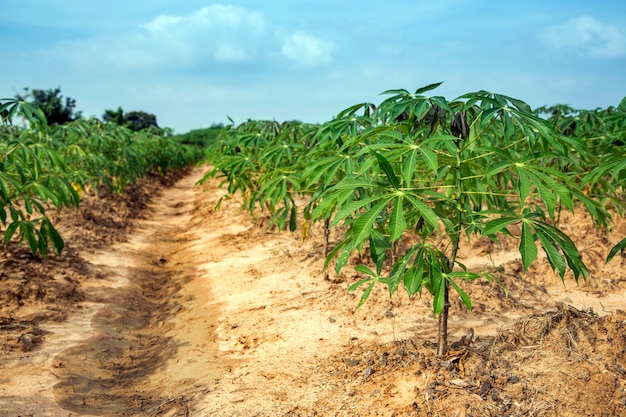This image captures a perspective from ground level, showcasing rows of verdant vegetation, likely tobacco plants, growing in light brown soil. The plants, adorned with large green leaves interspersed with hints of yellow, are arranged in two long, parallel rows separated by a shallow, moist trench. The scene extends into the distance, emphasized by the depth and angle of the photograph, making the rows appear to stretch endlessly. In the bright, vibrant background, a stunning blue sky adorned with fluffy white clouds adds a serene atmosphere. The vibrant green of the foliage contrasts beautifully with the brown soil, creating a vivid and detailed landscape. The overall perspective, from a low vantage point, enhances the viewer's immersion into this agricultural setting.